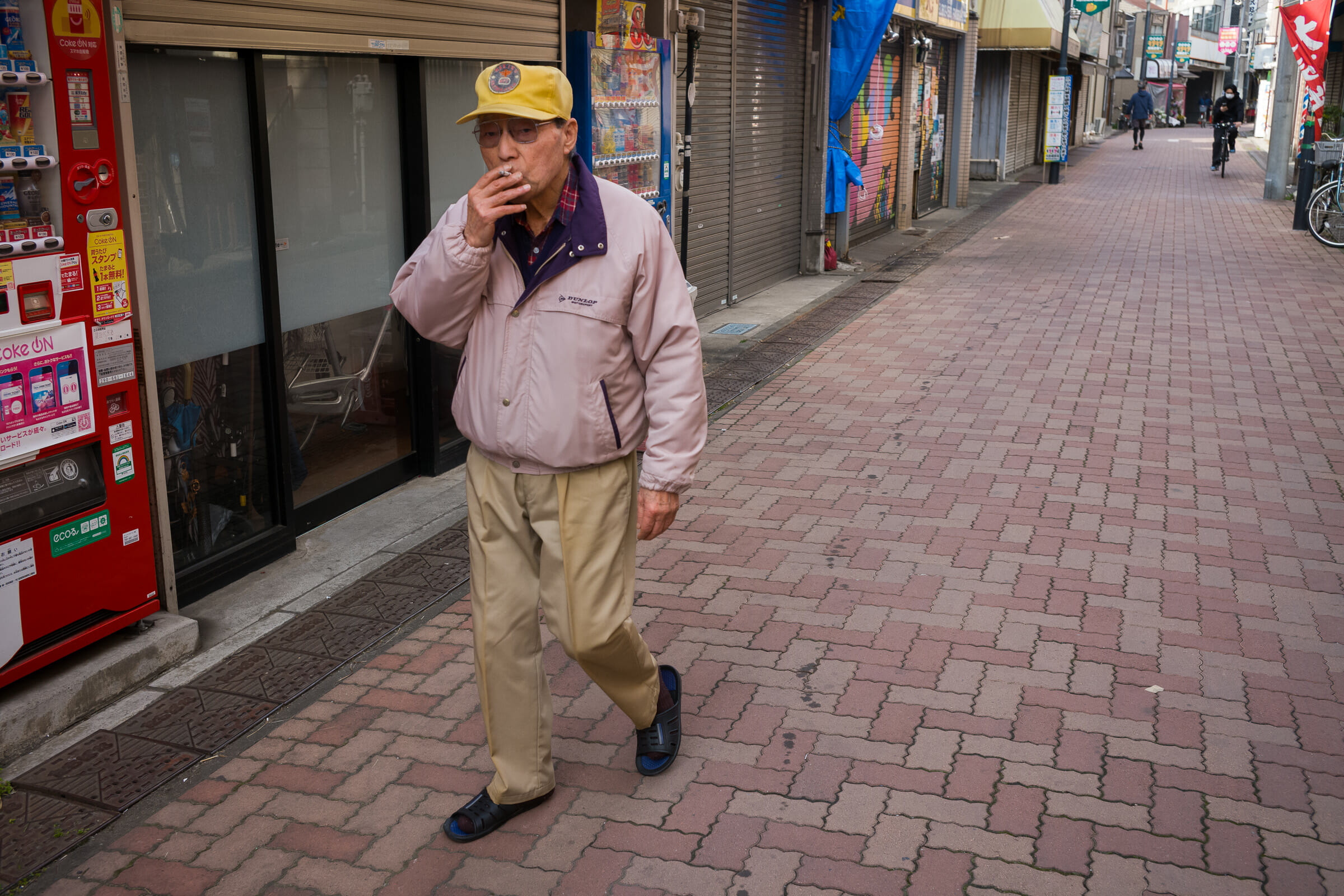The image captures a quaint, clean, brick-paved street in an older, possibly European or Asian city. The street is narrow and looks more like an alley, with buildings lining both sides, many of which have closed storefronts covered by metal garage-like doors. The paving stones vary in shades of light and medium brown, giving the street a historical charm.

Central to the image is an older man, likely in his mid-60s, who is smoking a cigarette. He is wearing glasses and a distinctive outfit: a light pink windbreaker or bomber jacket with a darker inner lining, light brown khaki pants, and black shoes or sandals. On his head, he sports a yellow baseball cap with some sort of logo on the front. His gaze is directed towards the camera as he walks down the street. 

To the left of the man, there's a vending machine positioned against one of the shut shops. In the background, the street stretches out with additional figures—two small, distant people who appear to be walking and another person riding a bicycle towards the camera, possibly wearing a face mask. The overall atmosphere is quiet and somewhat deserted, suggesting it might be during a period when businesses are closed, possibly hinting at the pandemic.